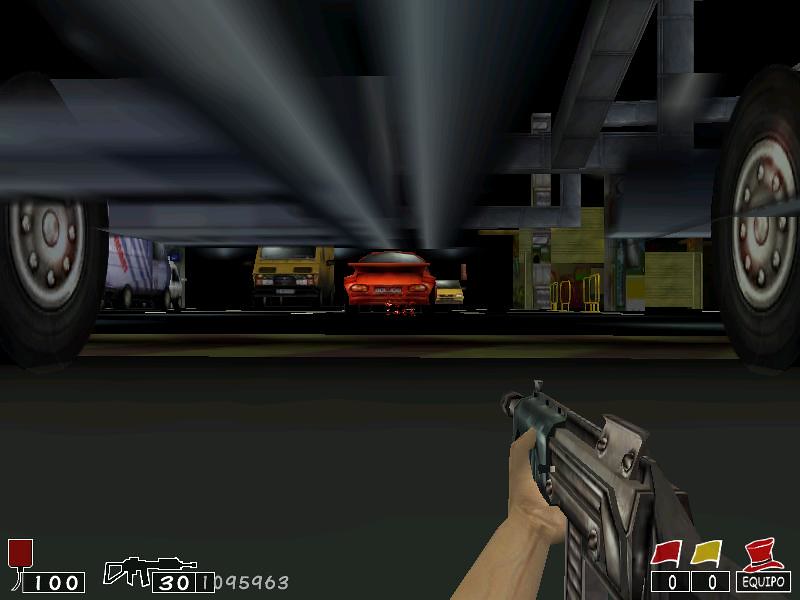A detailed image description of a screenshot from a first-person shooter game features the player lying prone beneath a car, the tires visible on both sides of the screen. The ground, which appears to be tar due to its black color, supports the player's perspective as they aim forward. At the center of the screen, a red car dominates the scene, with additional vehicles—a yellow van to its left, a white truck further left, and a small yellow car behind it to the right—creating a cluttered urban environment.

The visual interface includes various HUD elements: in the bottom left corner, a red block displays the number "100" in white within a rectangular outline, indicating health or armor status. Below it, an icon of a semi-automatic weapon, with its butt facing left and barrel pointing right, shows the number "30" beneath it, likely representing the current ammunition count, accompanied by additional pale gray numbers.

In the bottom right corner, a red flag above an outlined black box with the number "0," a yellow flag above a "0," and a red top hat labeled "Equipo" indicate team scores and status. The first-person perspective allows the player to see their character's left arm and hand gripping the semi-automatic weapon, from the edge of the butt to the barrel. This immersive angle underscores the intense, action-oriented gameplay environment.